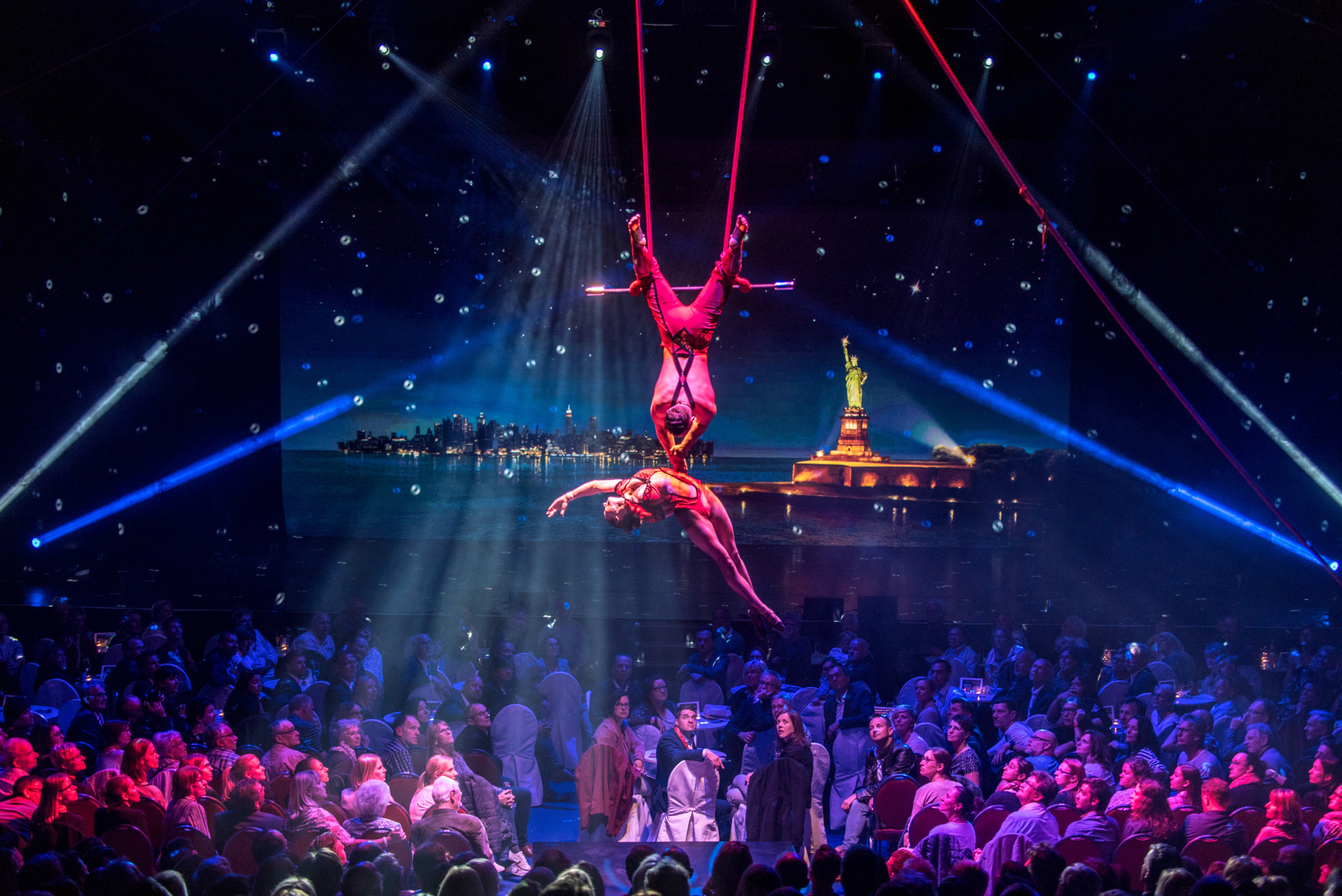This photograph showcases a mesmerizing performance inside an expansive hall, bustling with an audience captivated by the spectacle. The hall is dimly lit, accentuated by a vibrant color theme of pink and blue lights. Suspended in mid-air, two acrobats perform an intricate aerial routine. The male acrobat, dressed in pink pants, securely holds the female acrobat, who is adorned in a striking red dress. They are both suspended by delicate pink ropes. Below them, the audience—a mix of standing and seated spectators—gaze upwards in awe. Adding to the dazzling display are scattered laser lights that vary in color, including blue and green. In the background, a large screen projects an evocative image of the Statue of Liberty, with an island and the cityscape beneath a sky brightened by scattered stars, enhancing the scene's dramatic ambiance.